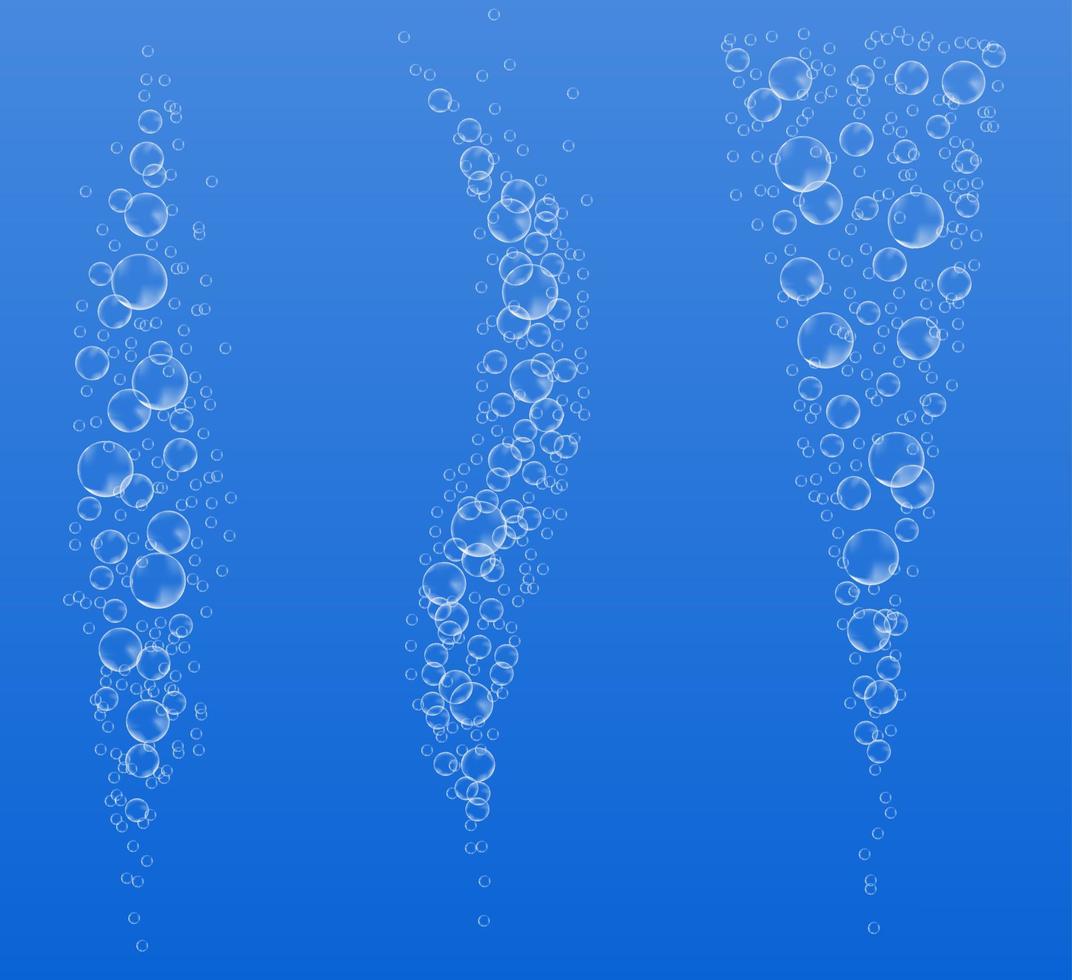This image features a gradient blue background, lighter at the top and darker towards the bottom, with three distinct columns of white bubbles arranged vertically. On the left side, the bubbles form a straight column, exhibiting a mix of sizes with some of the largest in the middle section. The central column of bubbles curves gently, almost like an S or a banana shape, again showcasing a variety of bubble sizes, particularly larger ones in the middle. The third column on the right follows a cone-like or pizza slice shape, narrowing to a point at the bottom and expanding outward as it ascends. This column also contains bubbles of varying sizes, with a notable concentration of larger bubbles in the middle section.